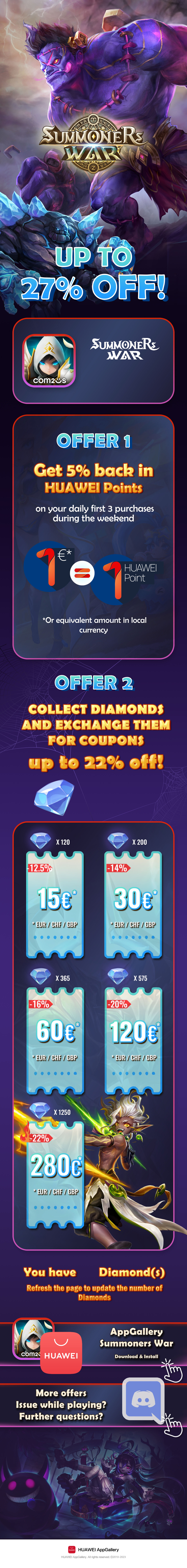The image appears to be a slightly blurred screenshot of a Discord or gaming-related page. At the very top of the page, there is a figure resembling a male or creature with a gold emblem, although the blurriness makes it difficult to discern details. Below this, bold blue text displays "27% off." Accompanying this are various icons and buttons.

There is a small square icon near the offer section. Following this, there are two offer buttons labeled "Offer 1" and "Offer 2" in blue. The page also displays a series of blue boxes with different numerical values: 15C, 60C, 280C, 30C, and 120C. In the bottom right-hand corner, a Discord button is recognizable, featuring the familiar white marshmallow-like figure set against a purple background.